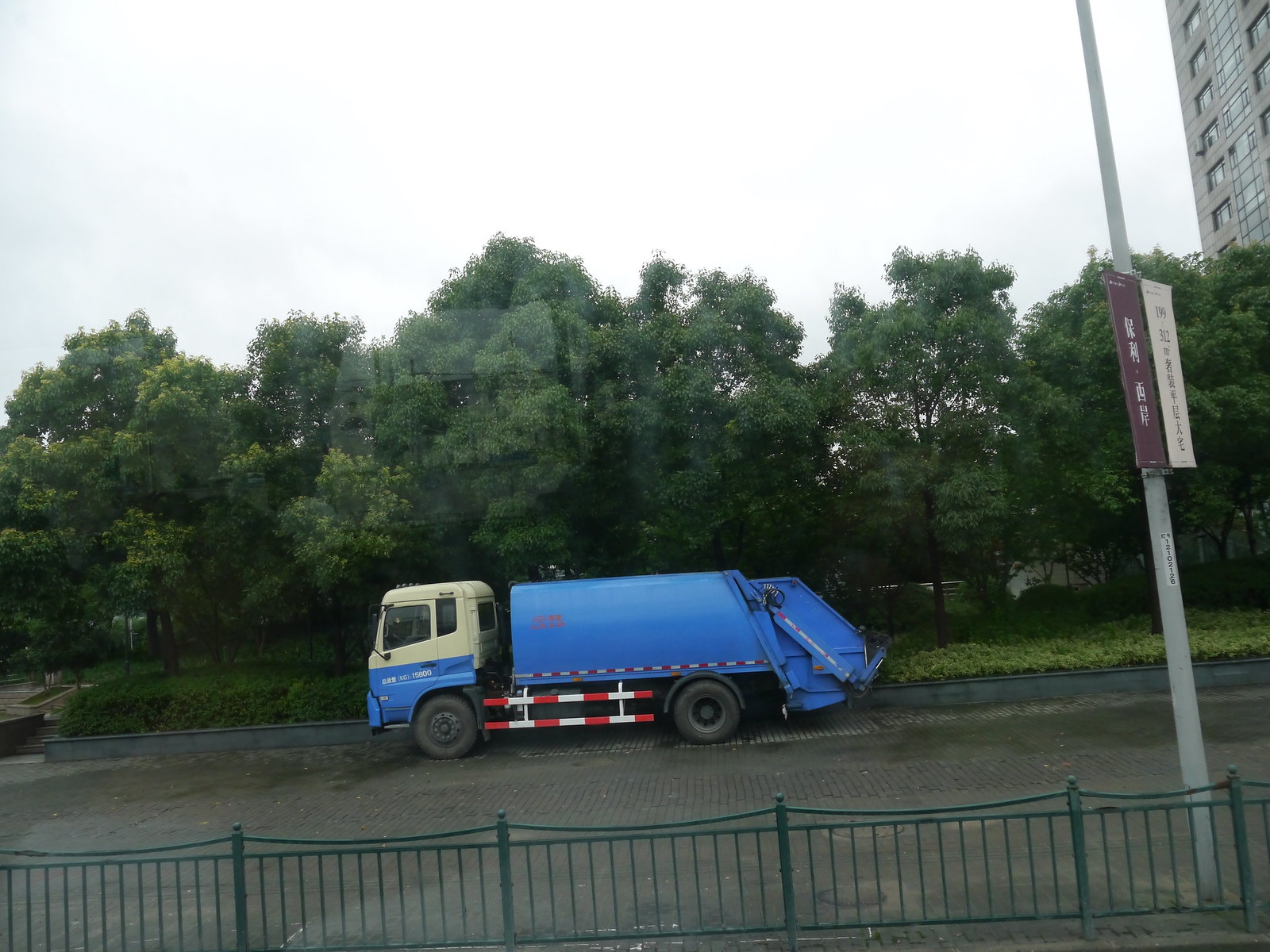This color photograph captures a compact, low-profile garbage truck on a city street next to a high-rise building. The truck features a distinctive two-tone cab-over design with a turquoise blue body and an off-white, yellowish top. Red and white striped supports are visible on its sides. Parked on a gray road, the truck is accompanied by a gray metal fence in the foreground and a line of trees with dark green leaves in the background against an overcast, light gray sky. A sign with Japanese writing on a post is also visible in the foreground. The high-rise building, likely an office structure, stands dominantly to the right of the image.